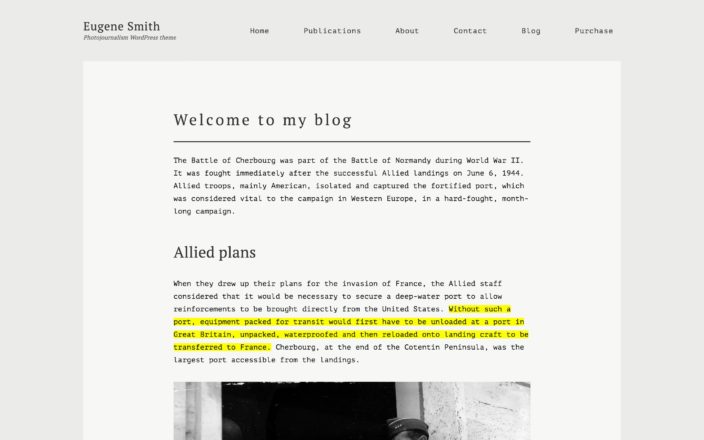This image is a partially cropped screenshot from a website with a light gray background on the left, right, and top borders. The top section features the name "Eugene Smith" in black print, with both 'E' and 'S' capitalized. Below the name, there is some small and blurred text. The navigation bar includes options for "Home," "Publications," "About," "Contact," "Blog," and "Purchase."

Within the central, bordered white background of the page, a bold headline reads "Welcome to my Blog," followed by a detailed paragraph in black text. The paragraph provides a historical summary of the Battle of Cherbourg, part of the larger Battle of Normandy during World War II. It details the events beginning with the Allied landings on June 6, 1944, leading to the American troops' isolation and capture of the fortified port of Cherbourg, a critical asset for the campaign in Western Europe. Further, it describes the Allied plans which emphasized the necessity of securing a deep-water port for direct reinforcements from the United States. Without such a port, logistical operations would have been significantly more complicated, requiring equipment to be unloaded in Great Britain, processed, and transferred to France.

A portion of this text, specifically from "Without such a port, equipment packed for transit would first have to be unloaded at a port in Great Britain, unpacked, waterproofed, and then reloaded onto landing craft to be transferred to France," is highlighted in yellow, resembling a marker’s color. 

The screenshot also includes an image displaying part of a wall and doorway, with the top of a person’s head in a hat partly visible, but the rest of the person’s head is cut off.